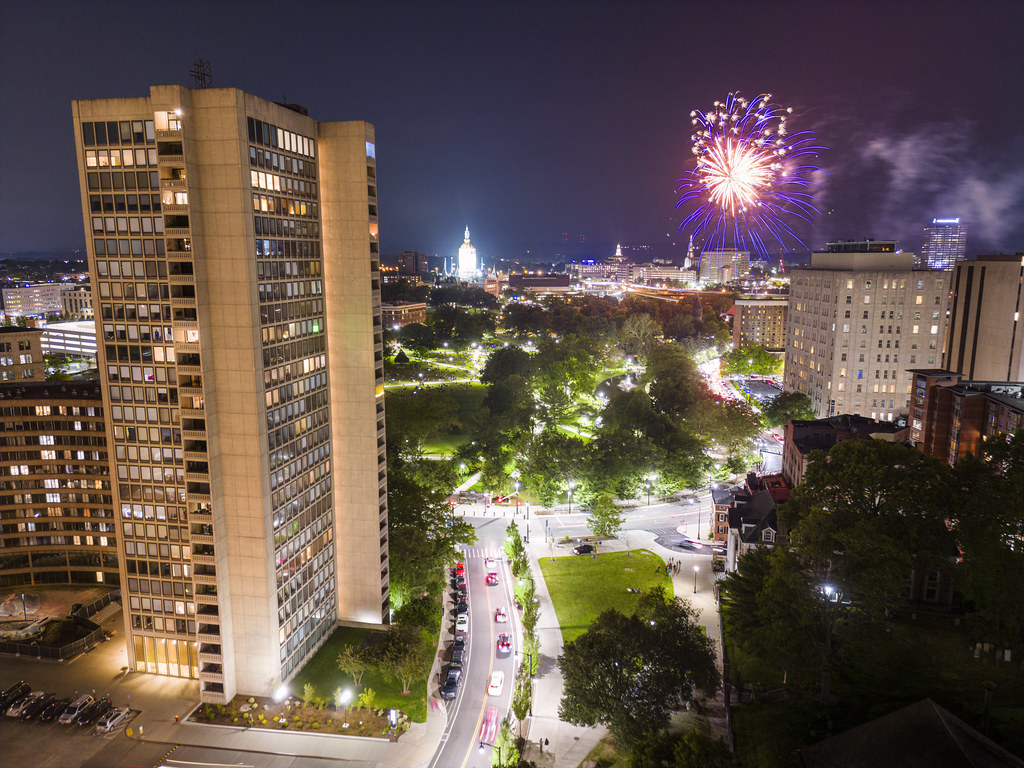This nighttime aerial photograph captures a bustling cityscape, possibly in the United States or Europe, illuminated by a spectacular fireworks display. The scene is marked by several tall buildings, one particularly prominent high-rise in the front left and another sizeable building to the right. Nestled among these structures is a large central park, surrounded by green trees and encircled by roads, adding a touch of nature to the urban environment.

The photograph reveals numerous cars parked around the tall building and along adjacent streets, suggesting a busy evening enhanced by the celebratory atmosphere. Another striking element is a brightly lit structure with a white, pointy top in the background, though its identity is unclear.

Highlighting the festive scene are the dazzling fireworks lighting up the dark blue sky, with colorful bursts of white, pink, and blue, accompanied by twinkling stars. The vibrant explosions and the widespread city lights create a lively and illuminated landscape. This image likely depicts a 4th of July celebration or a similar festive event, showcasing the city's bright and communal spirit.